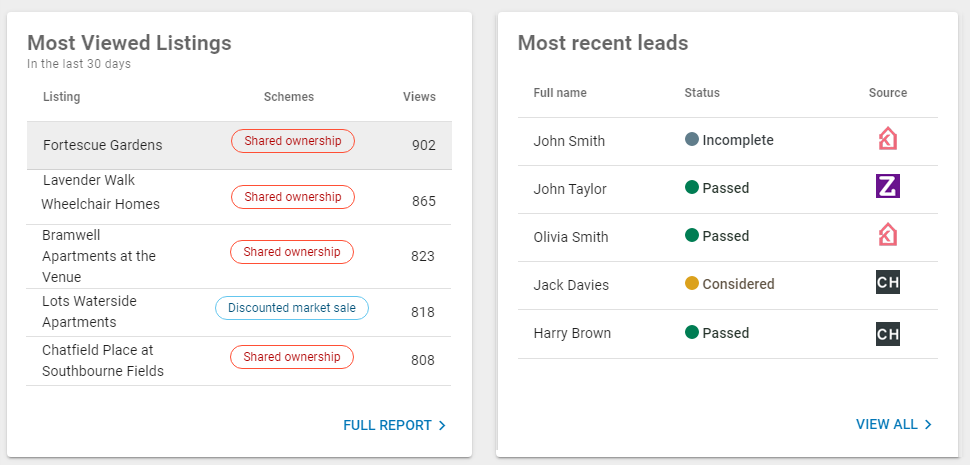This detailed image caption represents two segmented visuals combined into a collage. The first section, titled "Most viewed listings in the last 30 days," displays a tabular format with columns for listings, schemes, and views. Notable listings include: 
1. Fortescue Gardens, shared ownership, with 902 views.
2. Lavender Walk Wheelchair Homes, shared ownership, with 865 views.
3. Bramwell Apartments at the Venue, shared ownership, with 823 views.
4. Waterside Apartments, discounted market sale, with 818 views.
5. Shedfield Place at South Bonfields, shared ownership, with 808 views.

The section concludes with an option for a full report.

The adjoining segment is labeled "Most recent leads" and features columns for full name, status, and source:
1. John Smith, status: incomplete, indicated by a navy blue circle and a house icon.
2. John Taylor, status: paused, marked with a green circle and a purple square housing the letter 'Z'.
3. Olivia Smith, status: paused, identified by a darker green circle and a home icon.
4. Jack Davis, status: considered, denoted with a yellow circle and a black square with 'CH'.
5. Harry Brown, status: paused, represented by a green circle and the 'CH' icon in black.

At the bottom, the segment offers a "View all" option for further details.